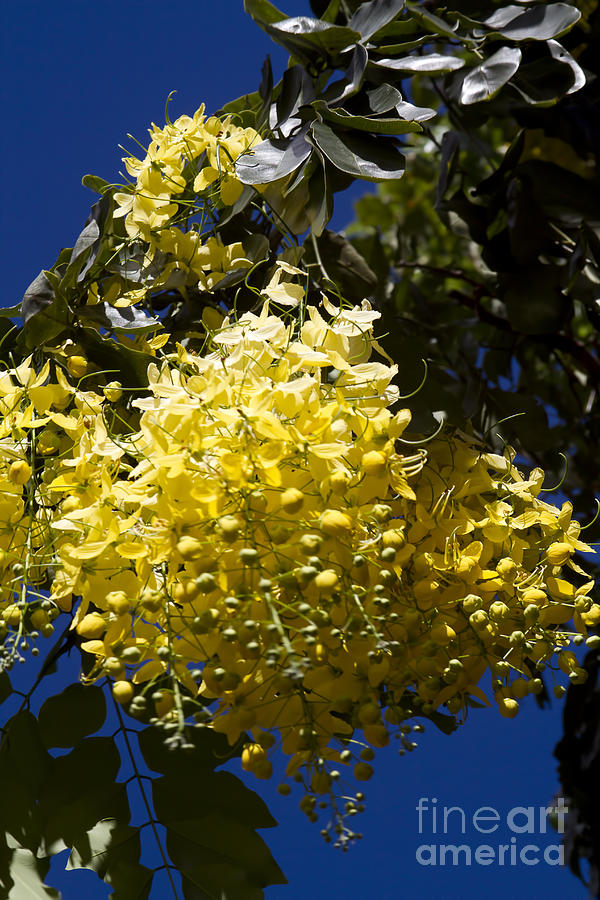This is a detailed and professional-looking color photograph with the words "Fine Art America" inscribed in the bottom right-hand corner. The image features an up-close shot of a flowering plant against a very dark blue sky. The plant showcases bright yellow flowers, which resemble honeysuckles with their protruding stamens and tiny buds, creating the illusion of a larger cluster of flowers. The leaves, which appear rubbery and fern-like, are dark green and some are hanging down in the foreground. In the background, additional blurry leaves can be seen, adding depth to the image. The photograph does not include any insects or other items, emphasizing the beauty of the flowers and the clarity of the sky.